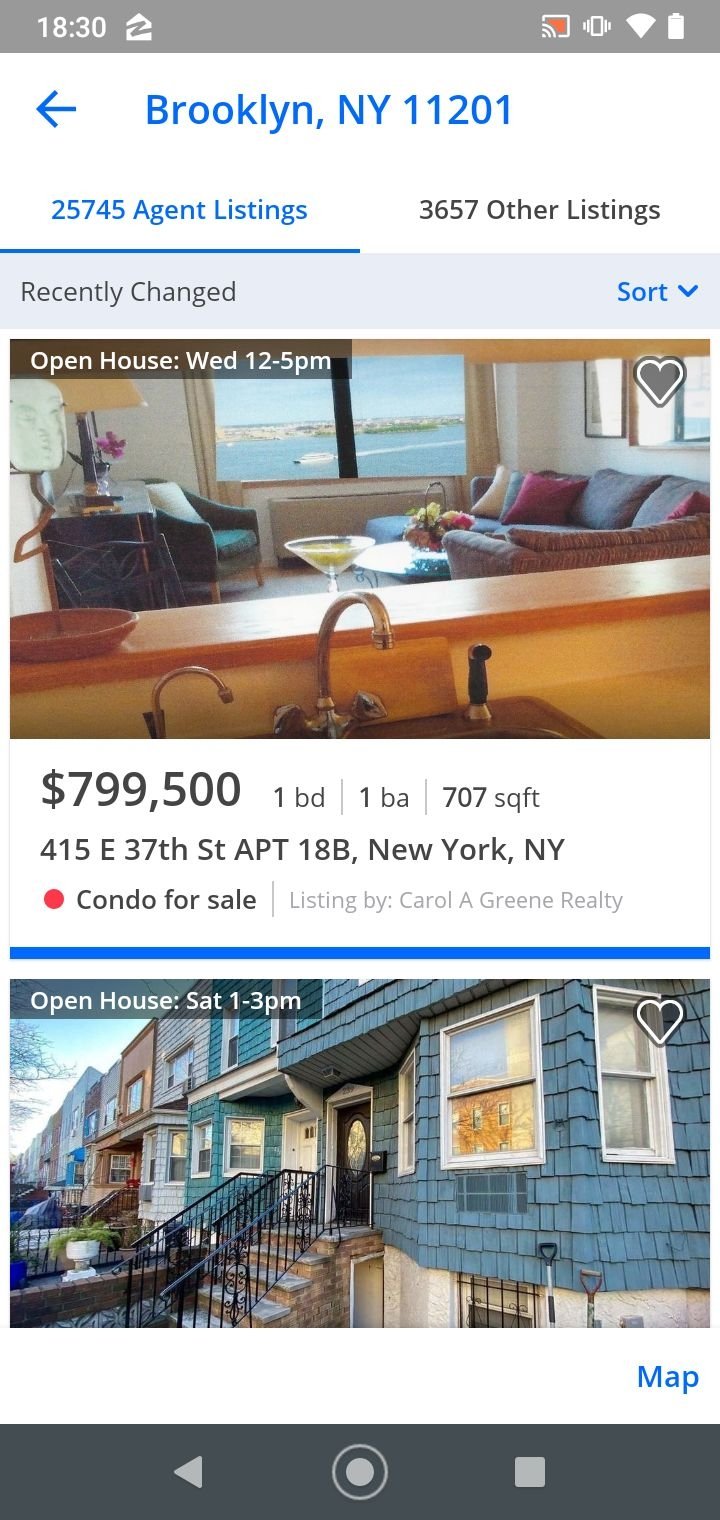Screenshot from a mobile phone depicting a real estate listing interface:

- **Top Bar:**
  - Gray bar with white font on the left displaying "18:30".
  - Small triangle icon with a gray "Z", Share screen icon, Vibration icon, Wi-Fi signal icon, and battery icon.

- **Listing Information:**
  - Large blue font at the top reading "Brooklyn, New York 11201".
  - Below in blue font, underlined: "25,745 agent listings".
  - To the right in gray font: "3,657 other listings".

- **Sorting Section:**
  - Light blue rectangle with black font stating "Recently changed".
  - On the right end: "Sort" in blue with an arrow pointing downwards.

- **Property Image:**
  - Photo depicting the interior of an apartment, seemingly taken from the kitchen area, looking over an island with a faucet.
  - Visible small living room with a gray couch and a window with a beach view outside.

- **Price and Details:**
  - Displayed below the image: "$799,500".
  - Further details: "1 bedroom, 1 bath, 707 square feet".